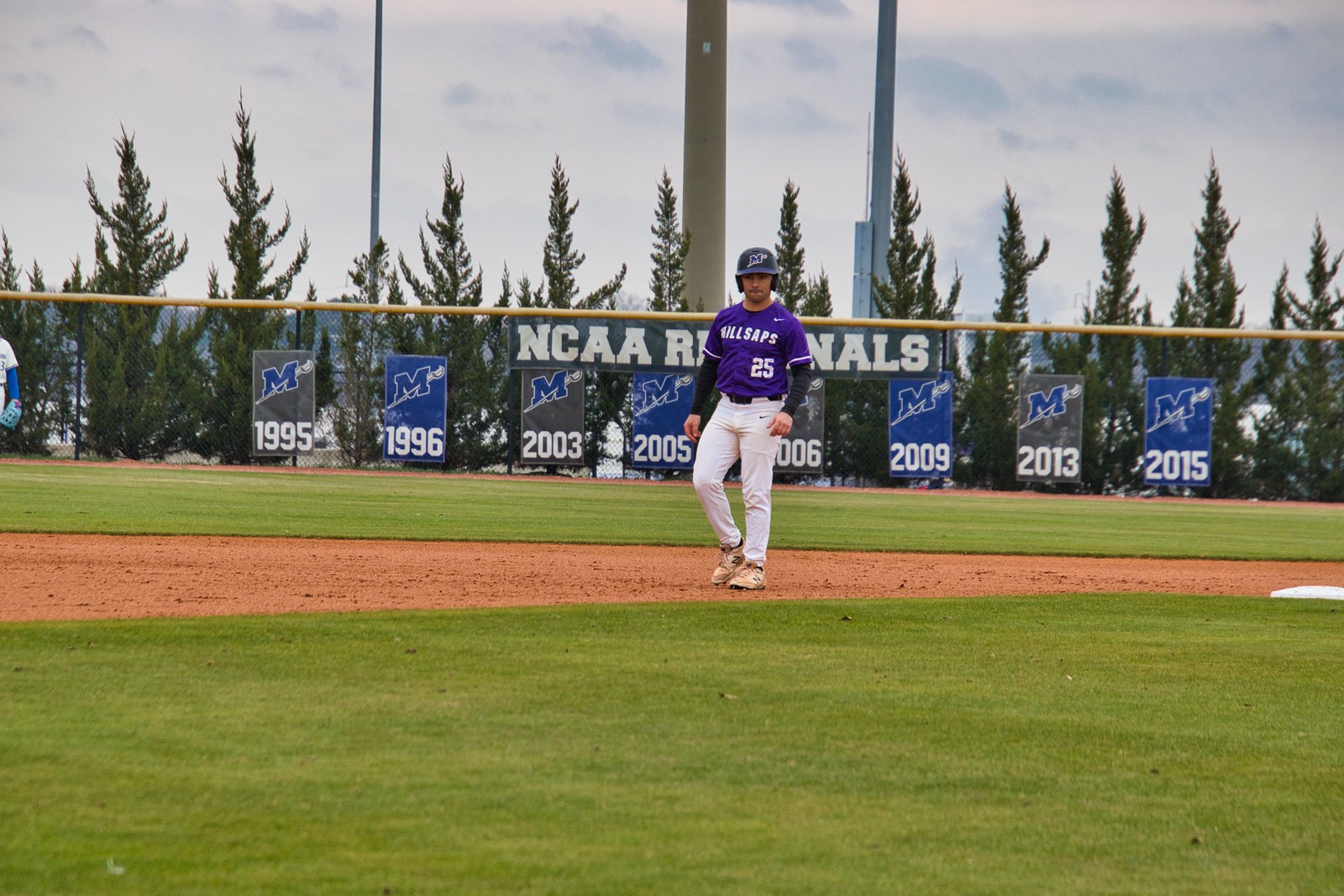A likely baseball player is seen here wearing white, long pants, a short-sleeved purple jersey with the number 25 displayed low down, and a long-sleeved black shirt underneath. He also dons a gray cap. The player appears to be taking a few steps away from a base, situated to the far right. The baseball field features neatly mown green grass, with a maintained dirt section visible in the middle. The outfield, in the far distance, is marked by the green grass and a wall adorned with NCAA banners. Beyond the outfield fence stands a row of large fir trees. All these elements suggest that this photo is captured during a baseball game.